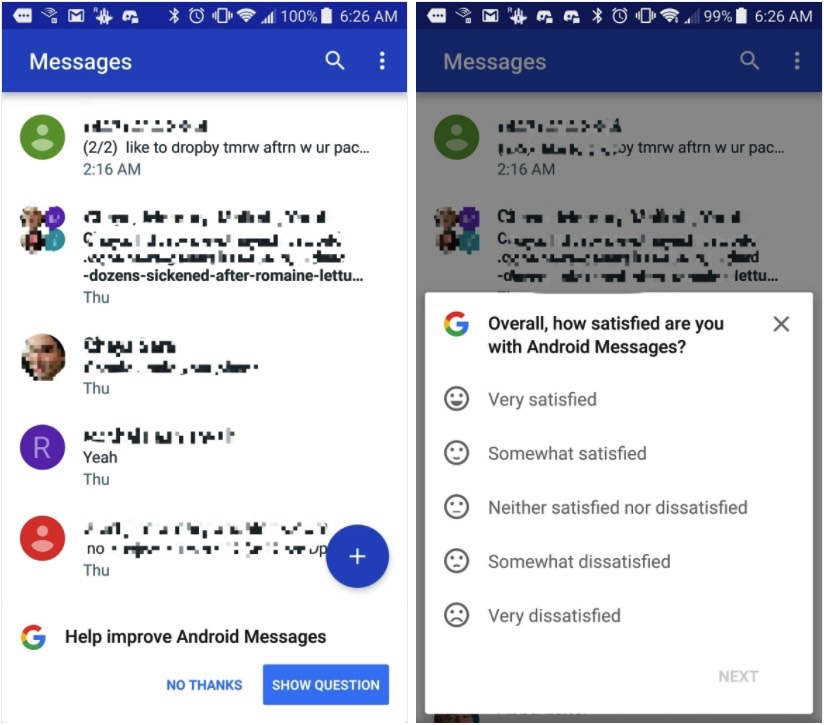Here are two screenshots captured from a smartphone, taken at 6:26 a.m. with a full battery charge. Both images display the messaging app, providing a clear view of its interface, including symbols for Gmail, Bluetooth, Wi-Fi signal, and more. 

### Left Image:
- **Header Icons:** Includes the magnifying glass for search and three dots for additional options.
- **Messages List:**
  - Several names are blurred out, indicating a focus on privacy.
  - One message thread visible reads "2 out of 2: like to drop by tomorrow afternoon with your pack and..." sent at 2:16 a.m.
  - A group text message is noticeable, having four different icons. One message links to "romaine lettuce," suggesting it was posted in the group chat on a Thursday.
  - Another thread only shows a blurred-out name with an unreadable message, indicating it was also sent on Thursday.
  - A single message simply says, "yeah," sent on Thursday.
  - Another message reads "no," sent on Thursday.
- **Footer Message:** The interface prompts the user with “Help improve Android Messages” and offers options for “No Thanks” or “Show."

### Right Image:
- **Feedback Section:**
  - A prominent box asks, "Overall, how satisfied are you with Android Messages?"
  - It provides a range of responses, from "Very satisfied," "Somewhat satisfied," "Neither satisfied nor dissatisfied," "Somewhat dissatisfied," to "Very dissatisfied."

These screenshots not only showcase the user's regular interaction with the messaging interface but also include an instance where user feedback is solicited to improve the app's performance. The details highlight common features such as text message timestamps, group chats, and feedback prompts designed to enhance user experience.